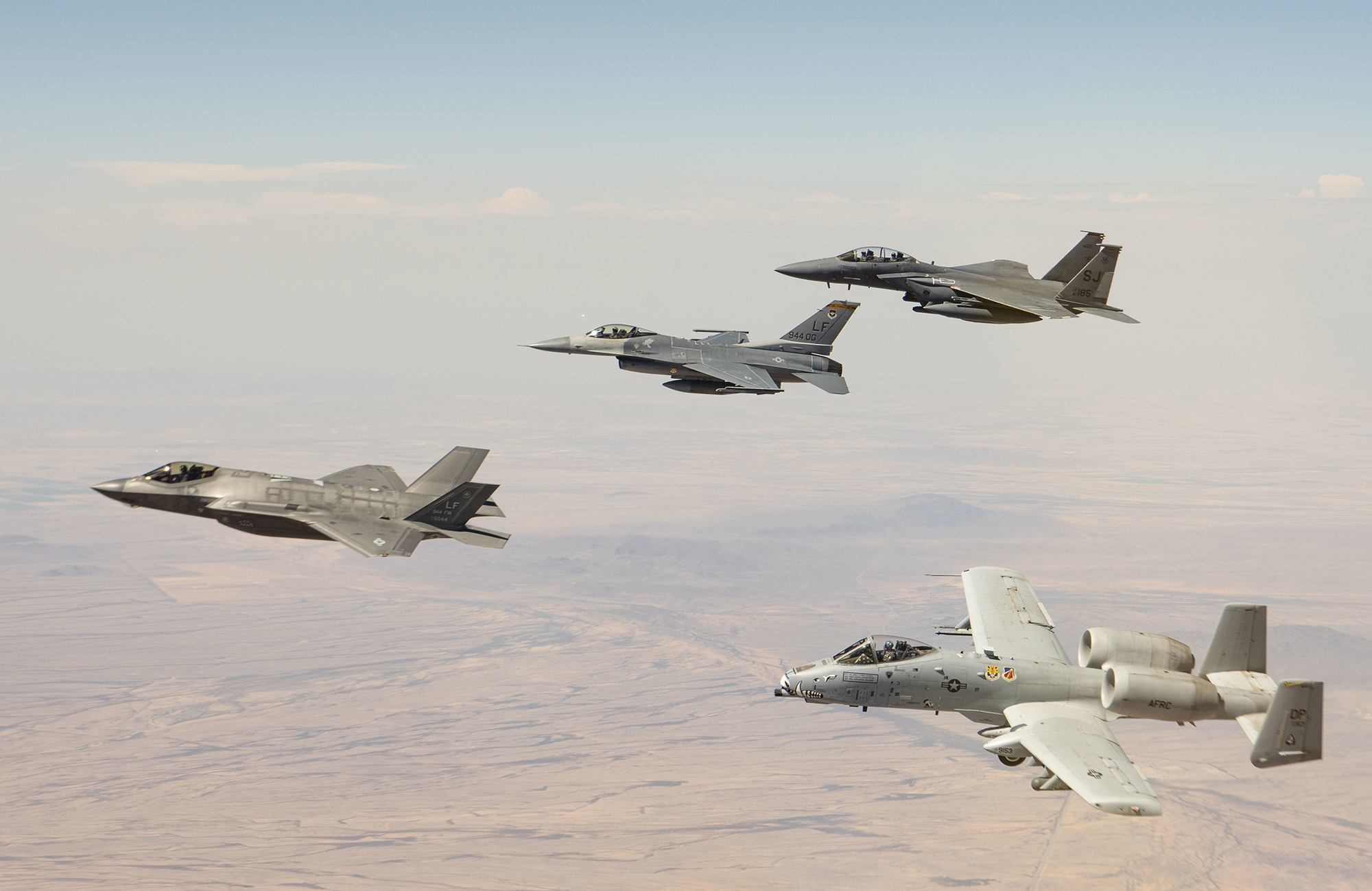This captivating midair photograph showcases four gray military aircraft flying towards the left against a backdrop of a blue, partly cloudy sky that gradually clears as it reaches the top. The ground below appears desolate, characterized by vast expanses of sand and dirt devoid of vegetation. Three of these aircraft are modern-day fighter jets, distinct yet similarly sleek and fast-looking, each designed to accommodate a pilot and a co-pilot seated in tandem cockpits. The fourth jet, different from the others in design, suggests an earlier era, possibly from the 1960s to 1970s. This unique aircraft, labeled as the DP AFRAC, has two engines positioned just before the tail and behind the wings, further indicating its age and style. Although the precise serial numbers or markings on the aircraft tails are not clearly visible, it's evident that among them, there are specific designations such as LF and SJ. The entire scene evokes a sense of aerial prowess and historical progression in military aviation.